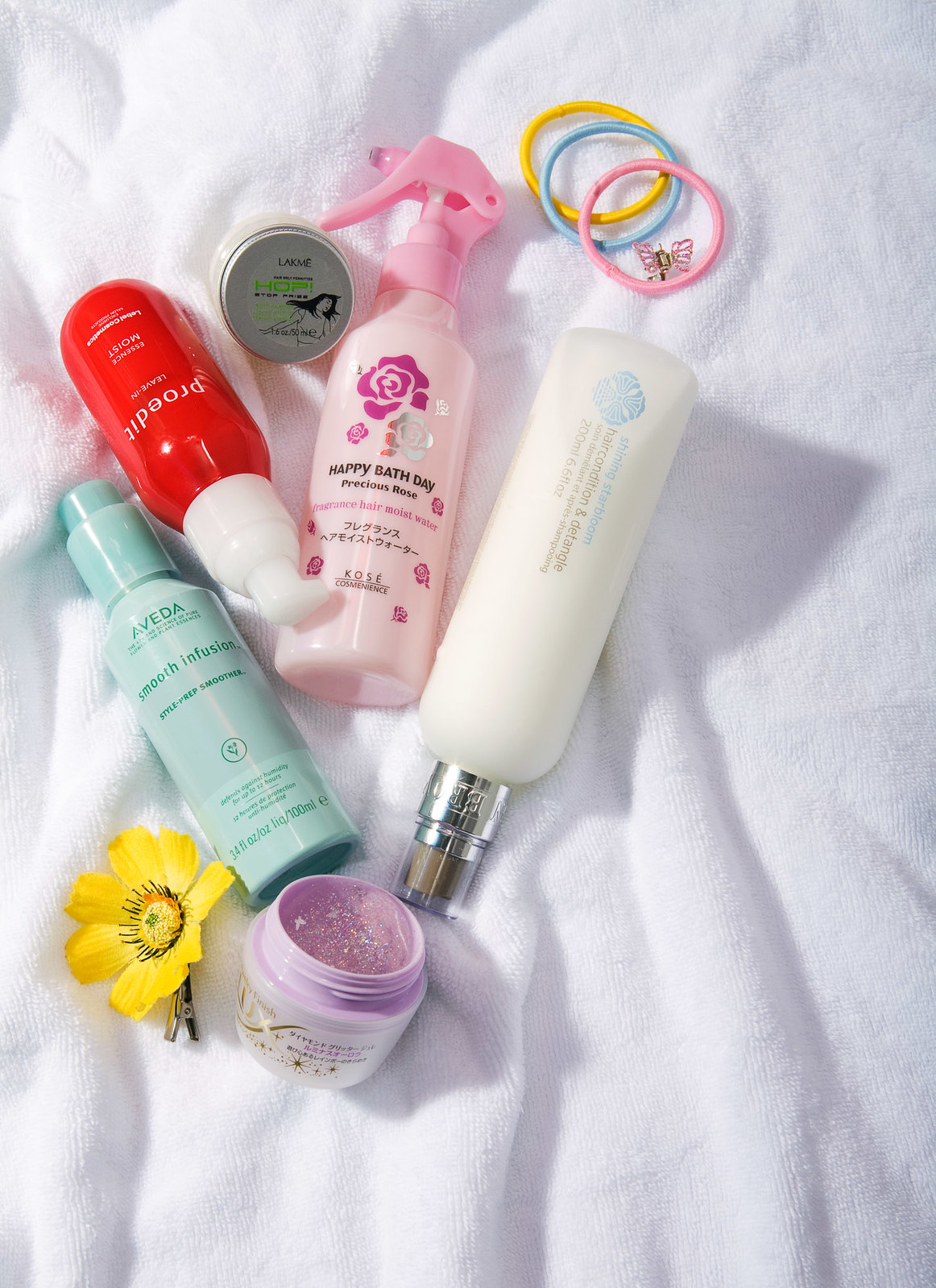This photograph showcases a neatly arranged selection of travel-sized beauty and personal care items, artfully displayed on a pristine white blanket or towel. At the forefront, a pink spray bottle labeled "Happy Birthday Precision Rose" suggests a fragrant body spray. Accompanying it, a sleek white bottle with a silver spray nozzle adds a touch of elegance to the collection. A red bottle with a white pump dispenser stands ready for use, exuding practicality and convenience.

Another prominent feature is a green bottle crowned with a green cap, labeled "Evita Smooth Infusion," hinting at a specialized hair product. Positioned at the top of the arrangement, three colorful hair ties—pink, blue, and yellow—offer a playful touch and practical utility. At the bottom, an open jar of sparkly lip gloss invites attention with its shimmering contents, complemented by a delicate yellow flower placed nearby.

This image is a delightful glimpse into someone's curated selection of essential beauty and hair care items, perfect for travel or daily use.